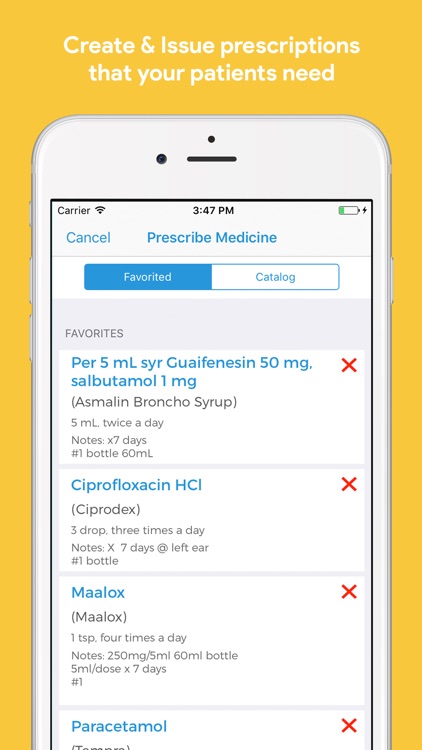The image is a detailed mock-up for a cell phone app designed for doctors to manage prescriptions for their patients. The background features a gradient of gold and yellow hues with text in white font at the top that states, “Create and issue prescriptions that your patients need."

Centrally, there is a depiction of a smartphone with a white bezel, slightly cut off at the bottom. The upper left-hand corner of the phone display indicates the network carrier and signal strength, suggesting connectivity. The time is shown as 3:47 p.m. in the upper center, while the battery indicator in the upper right-hand corner shows a low charge.

The app interface showcased on the phone screen features two tabs at the top labeled “Favorited” and “Catalog,” with the “Favorited” tab being active. Below these tabs is a list of medications marked as favorites, each neatly enclosed in white boxes.

The first listed medication reads: 

- **Per 5 ml**: S-Y-R, **Guaifenesin 50 mg**, S-A-L-B-U-T-A-M-O-L 1 mg
- **Brand Name**: (Azmalin, BronchoCere)
- **Instructions**: 5 milliliters twice a day
- **Notes**: X, 7 days, number one bottle, 60 ml

Further entries follow a similar format. 

This image effectively demonstrates the utility of the app by emphasizing its key features, such as ease of access to favorite prescriptions and detailed prescription management guidelines, all aimed at streamlining a doctor’s tasks in patient care.